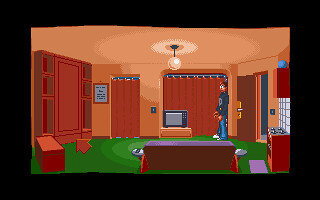The image is a detailed screenshot from a video game, depicting a basic animation of a living room, possibly in a hotel or residence. The outer border of the image is black, framing a room with tan-colored walls and green carpet. Dominating the left side of the room is a large brown cupboard with open shelves, next to which sits a brown bench or drawer. An arrow cursor points towards this cupboard, indicating it may be an interactive element. A picture frame hangs on the right of the cupboard, and brown curtains cover large windows, including a longer curtain behind a small TV that sits on a wooden stand. 

To the center right of the scene, a male figure stands wearing a dark blue long-sleeved shirt, blue jeans, and white shoes. Behind him, there's an open front door made of wood with a brass handle, revealing a dark night outside. A brown couch is positioned at the bottom of the image, facing the TV, with what appears to be a kitchen area on the right side, featuring a stovetop with a tiled backsplash. The room is lit by a white globe light fixture hanging from the ceiling. The overall setting is an animated, minimally detailed environment, emphasizing the interactive elements of the video game.